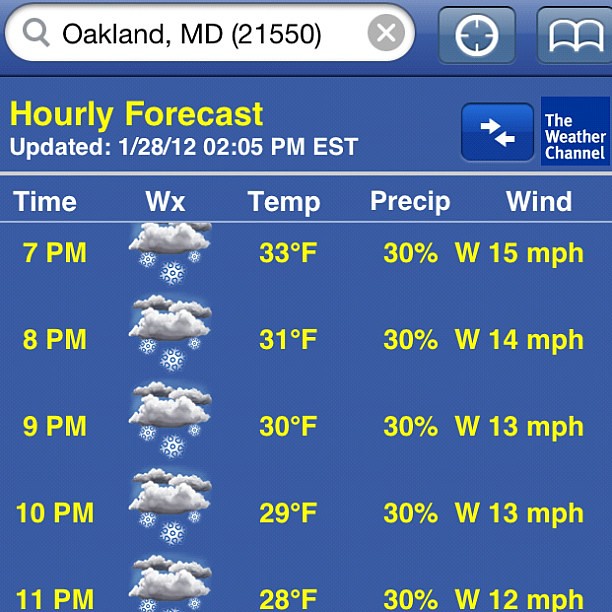This detailed screenshot captures a weather report for Oakland, Maryland, dated January 28, 2012, at 2:05 PM EST. The report is titled "Hourly Forecast" and is sourced from The Weather Channel. Displayed on a blue background with white and yellow letters and bordered by various icons, it presents precise weather predictions between 7 PM and 11 PM. The columns include headings for Time, WX (Weather), Temp (Temperature), Precip (Precipitation), and Wind. As the evening progresses, snowstorm conditions are anticipated, indicated by icons of clouds and snowflakes. Wind speeds start at 15 mph at 7 PM before decreasing to 12 mph by 11 PM. Temperatures drop from 33 degrees to 28 degrees, with a consistent precipitation probability of 30%. The comprehensive forecast suggests steady snowfall, potentially extending beyond 11 PM. The visual layout, including the blend of colors and icons, conveys a snowy evening ahead for Oakland, Maryland.